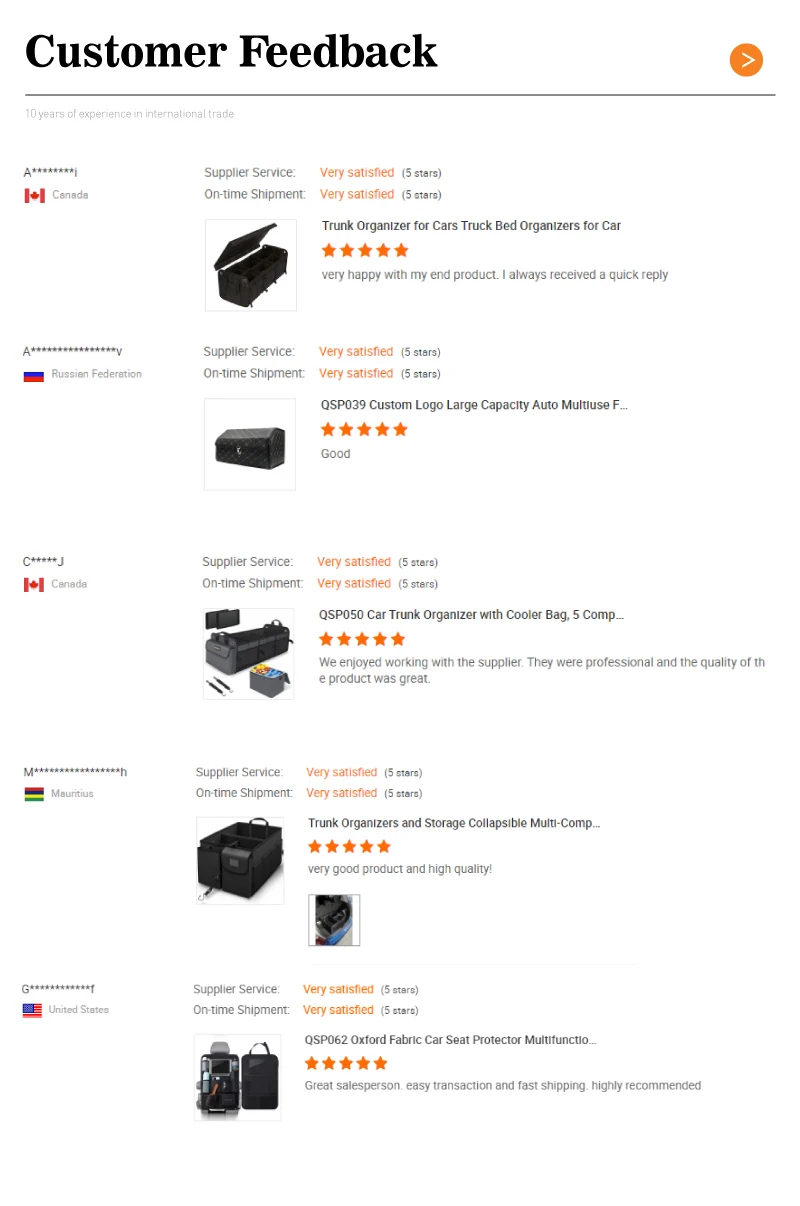This image showcases a customer feedback page on a website, specifically illustrating a detailed table with three columns labeled as follows: "Item," "Supplier," and "Service." The table lists five distinct items, each accompanied by a description and a five-star rating. The items under review include:

1. **Trunk Organizer for Cars/Truck Bed Organizer** – A versatile storage solution resembling a toolbox or storage box.
2. **Custom Logo Large Capacity Auto Organizer** – A high-capacity car accessory featuring a custom logo.
3. **Trunk Organizer Cooler Bag** – A multi-functional organizer that also serves as a cooler.
4. **Trunk Organizer and Storage Collapsible** – A collapsible storage unit, potentially identified as "Menu Camp."
5. **Backpack** – Though the description is less specific, it maintains the five-star rating consistency.

This layout allows users to quickly assess customer satisfaction and product details at a glance.